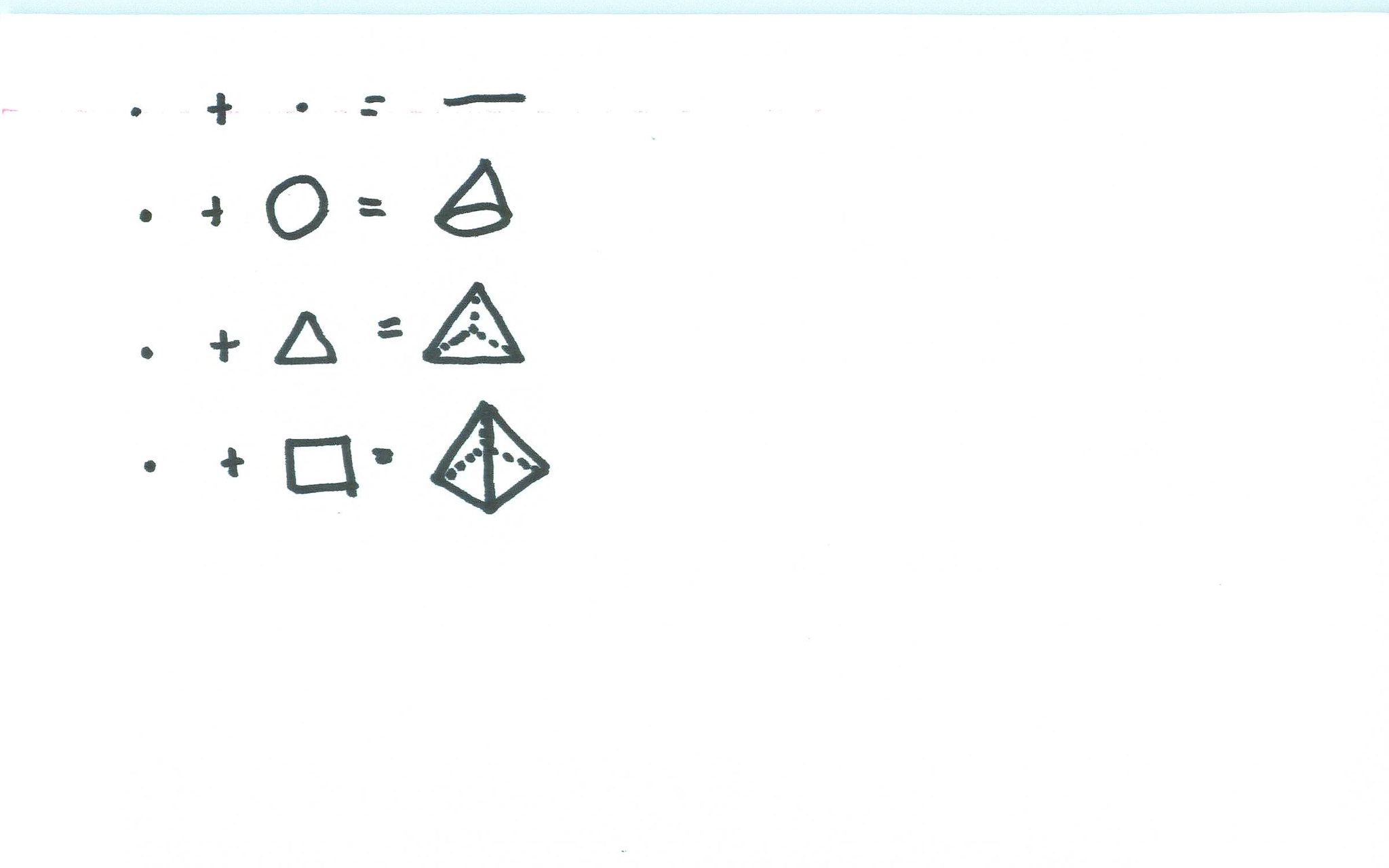A black marker illustration on a white background displays a series of geometric formulas arranged in four rows. Each row begins with a dot (.) followed by a plus (+) sign, with the third character in each line varying. The top row features "..+..=", demonstrating that a dot plus a dot equals a straight horizontal line. The second row shows "..+O=", indicating that a dot plus a circle results in a cone-shaped figure. In the third row, "..+△=" denotes that a dot plus a triangle yields a triangle with dotted lines extending from each vertex inward, converging at a central point. The fourth row presents "..+□=", representing that a dot plus a square forms a four-sided pyramid, with dotted lines illustrating the hidden edges and the obscured base.